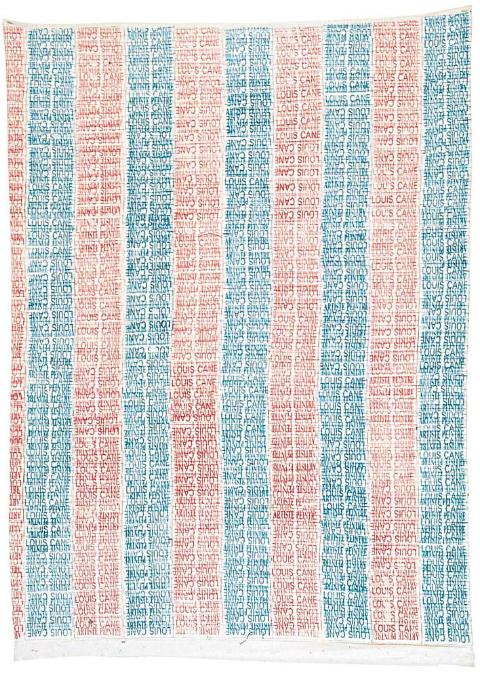The image showcases a rectangular piece of fabric, possibly a towel or tapestry, oriented vertically with a predominant white background. There are long vertical stripes of varying thickness running down its length. Starting from the left, it begins with a thin, light pink stripe, followed by thicker alternating stripes of a dark teal-blue and a rusty red color. This alternating pattern repeats nine times, consisting of thick stripes of color interspersed with thin white lines. Notably, each stripe appears to be comprised of words, though they are somewhat jumbled and hard to discern, seemingly forming the words "Lewis Kane." Both the top and bottom edges are bordered with a solid white section, enclosing the design.